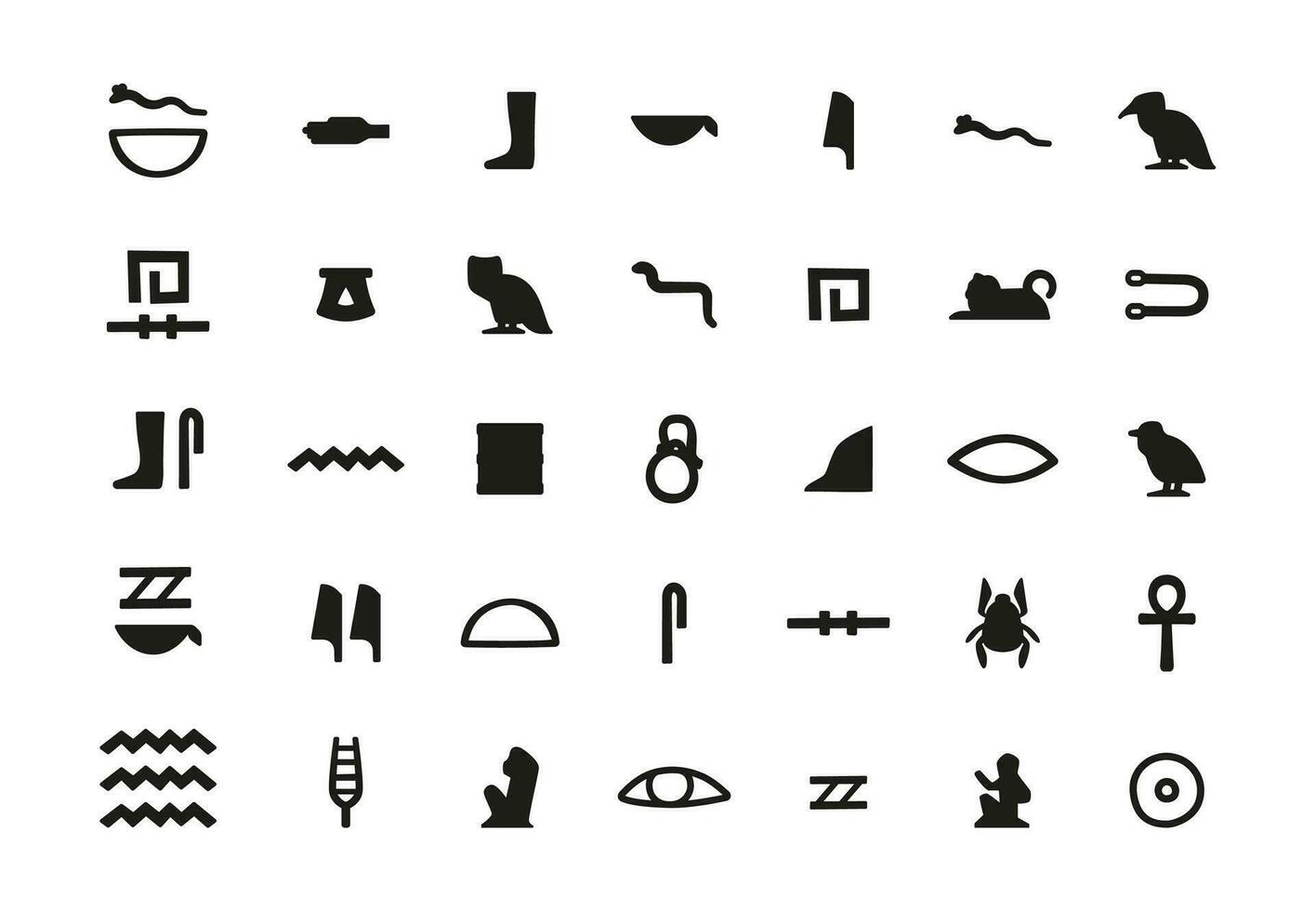The image features a grid of ancient Egyptian hieroglyphic symbols, arranged in five rows and seven columns, against a stark white background. Each black vector illustration depicts a variety of iconic Egyptian imagery, such as a dung beetle, an owl, a snake, and several birds. Other notable symbols include a simplistic eye without a pupil, a circle over a cross, a boot, a cane, and a series of parallel squiggly lines. The glyphs also feature a ZZ shape over a bowl, reinforcing the ancient thematic elements. This collection serves as an illustrative array of different hieroglyphic symbols rather than conveying a specific message.